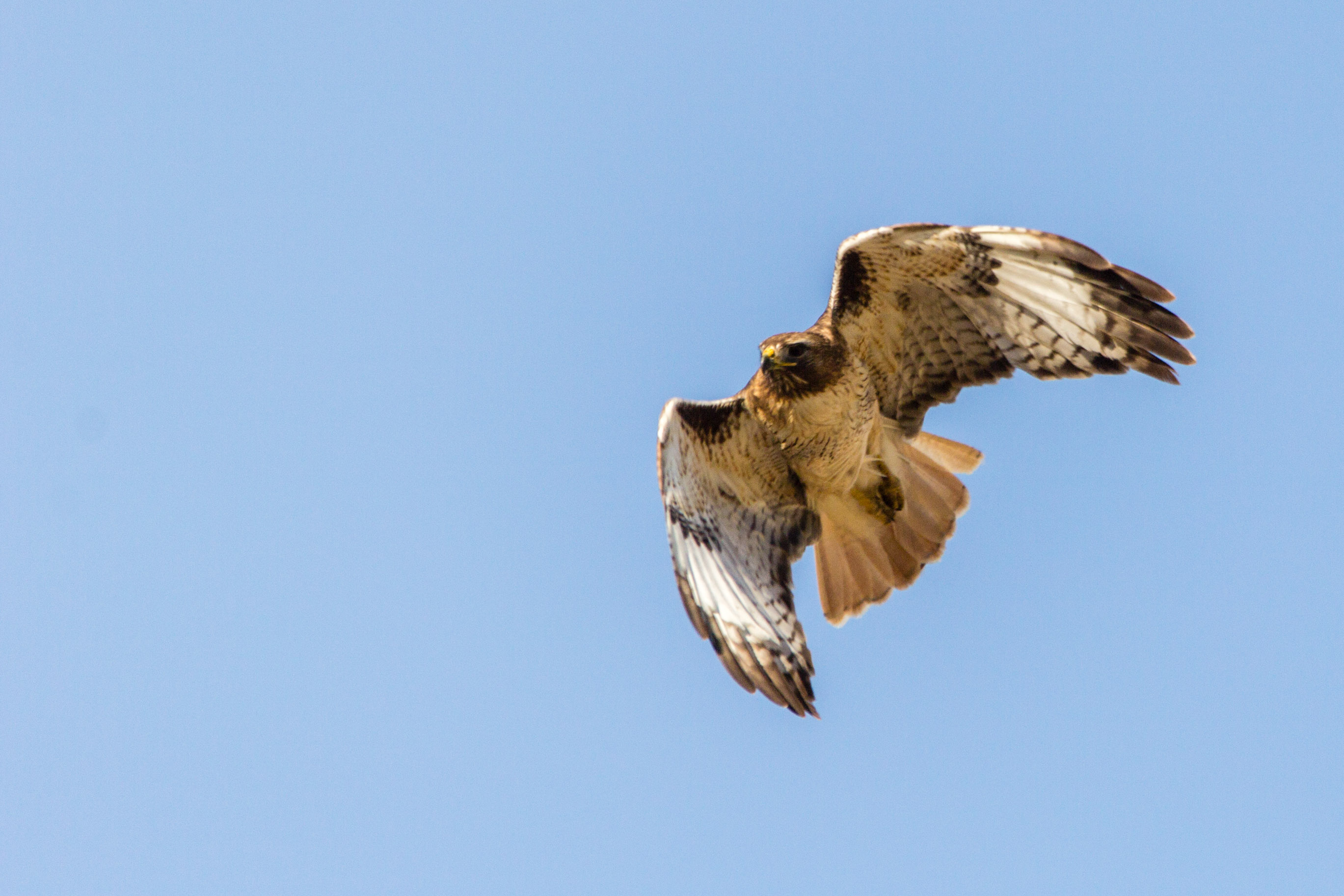Against a clear, cloudless, light blue sky, a medium-sized bird of prey is captured mid-flight. Its majestic wings are fully outstretched, showing off a striking contrast of white feathers interspersed with black markings, particularly prominent at the tips of the wings. The bird's shoulders and midsection exhibit a blend of light brown hues, with a subtle gradation towards darker brown tips. Its tail feathers are fanned out in a similar light brown shade, adding to the dynamic sense of movement. The bird, possibly a falcon or hawk (though some might mistake it for an eagle), has its talons folded tightly against its body and its beak is accented with a distinct touch of yellow. The intent focus in its eyes suggests it might have spotted something on the ground below, preparing to dive at any moment.